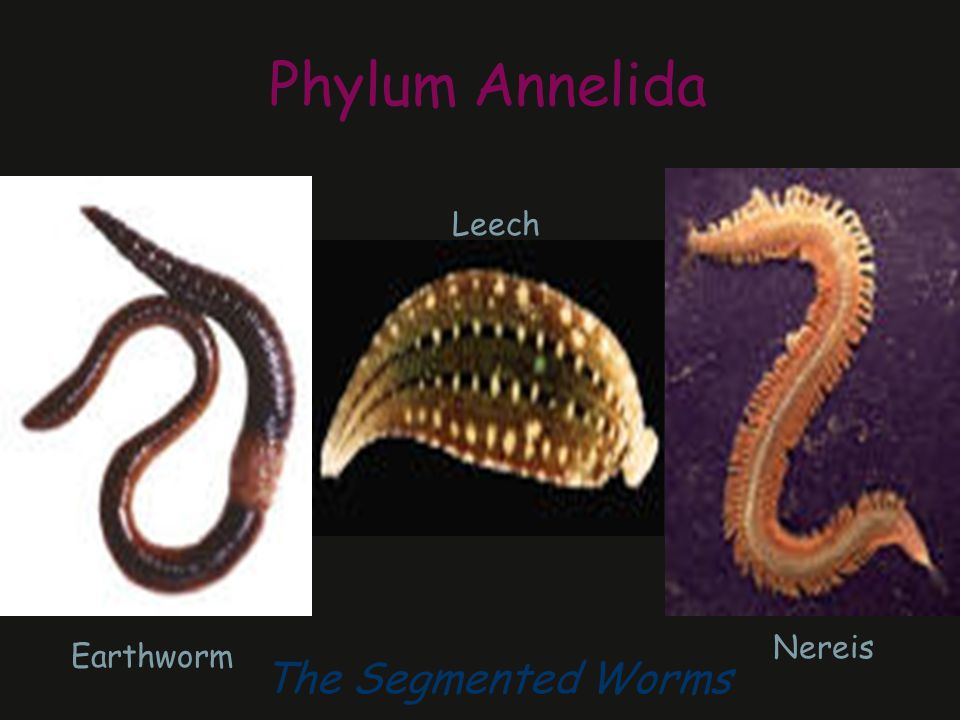The poster features a scientific illustration with a primary black background, reminiscent of a high school science project. At the top, in bright magenta letters, it reads "Phylum Annelida." Below this heading, there are three distinct sections featuring images of segmented worms. The left section, with a white background, displays a brownish-red earthworm labeled "earthworm" in light green text. In the center, on a dark blue or almost black background, a beige-colored leech is depicted, described as having a body with teeth-like structures. On the right side, against a purple-brick backdrop, there is an image of a Nereis, a centipede-looking creature with a yellow and orange coloration, arranged in a backward S-shape with visible feelers. At the bottom of the poster, in a barely readable muted blue font, the text "the segmented worms" is written, emphasizing the shared classification of these organisms.